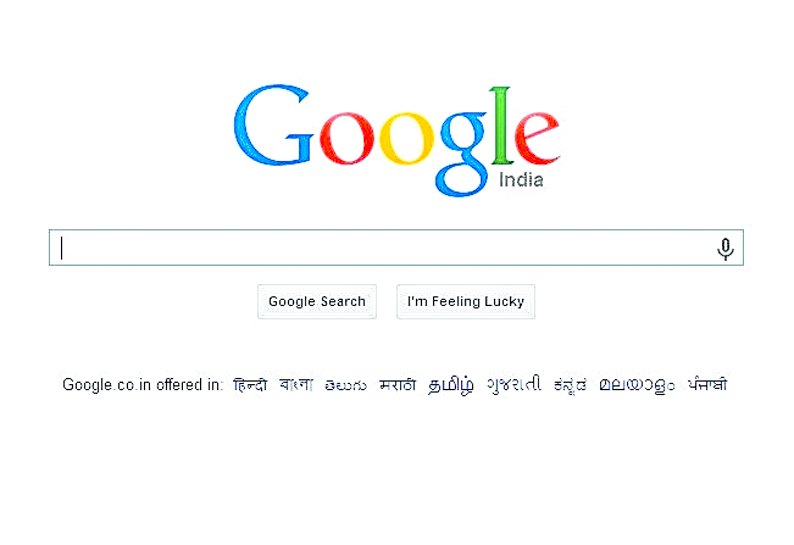The image depicts the homepage of Google India, as it would appear on a standard computer screen. Set against an all-white background, the central focus is the Google logo, which is prominently displayed in the middle of the page. The logo features the letters "G-O-O-G-L-E," with the "G" in blue, the first "O" in red, the second "O" in yellow, the lowercase "g" in blue, the "L" in green, and the "E" in red. Directly beneath the "L" and "E," the word "India" is written in black capital letters.

Below the logo is the search bar, which includes a small vertical line cursor on the left side and a microphone icon on the right side, indicating voice search capability. Underneath the search bar are two buttons: the "Google Search" button and the "I'm Feeling Lucky" button. Additional text at the bottom of the image includes the URL "Google.co.in" and an assortment of characters in a script that likely represents one of the many languages used in India. This further signifies that the webpage is specifically tailored for Indian users.